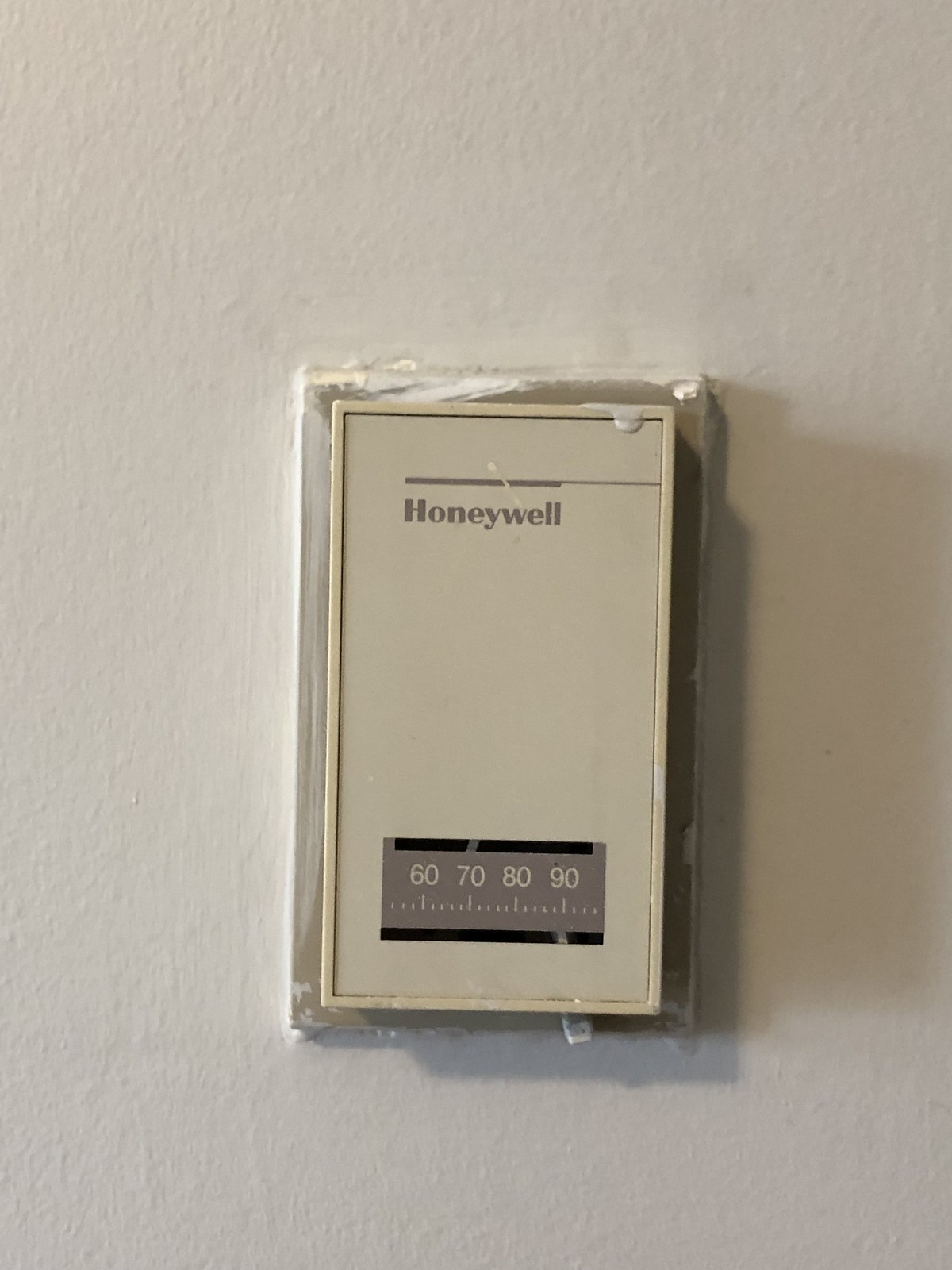The image depicts an old Honeywell thermostat mounted on a white wall. Centrally placed on the wall, the thermostat features a base with a grayish-brown, rectangular background that appears to have scattered patches of white paint, possibly due to wear or partial painting. The thermostat itself is slightly smaller than the base and has a light tan or beige hue. It is vertically oriented, taller rather than wider, with the word "Honeywell" inscribed at the top in brownish font, accompanied by a horizontal line extending from the text to the right edge of the device.

At the bottom part of the thermostat, there is a horizontal rectangular box in dark gray, containing white numerical markings: 60, 70, 80, and 90, which indicate temperature settings. Fine tick marks, both long and short, are positioned beneath these numbers to signify incremental temperature levels. A small white switch, located at the bottom of the thermostat near the 90-degree mark, is designed to slide left or right to adjust the temperature setting.